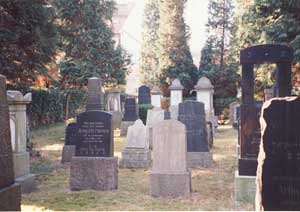This is a detailed photograph of a tranquil, sunlit graveyard, taken during the daytime in the fall. The cemetery features a mix of light green, dark green, and brown grasses, with areas of worn earth where visitors have walked. The scene is bordered by large, mature trees in varying shades of green and autumnal hues, along with a dark green hedgerow on the left side. The sky above is a pale blue, enhancing the serene atmosphere.

The gravestones vary significantly in size, from modest to towering, many reaching between four and seven feet tall. They are crafted from various materials, including light gray, dark gray, tan, black, and granite, some with intricate carvings and ornate details. Most of the headstones are rectangular with curved tops, while a few are more elaborate and ornate, featuring carved centers and resting on square or rectangular concrete pedestals.

In the background, there are three prominent pillars: two large ones with curved tops that are gray and white, and a third slightly obscured pillar. Additionally, some headstones appear quite old, with one particularly tall headstone in the foreground standing out. There is also a distant fence covered in shrubs, contributing to the peaceful, secluded feel of the cemetery.